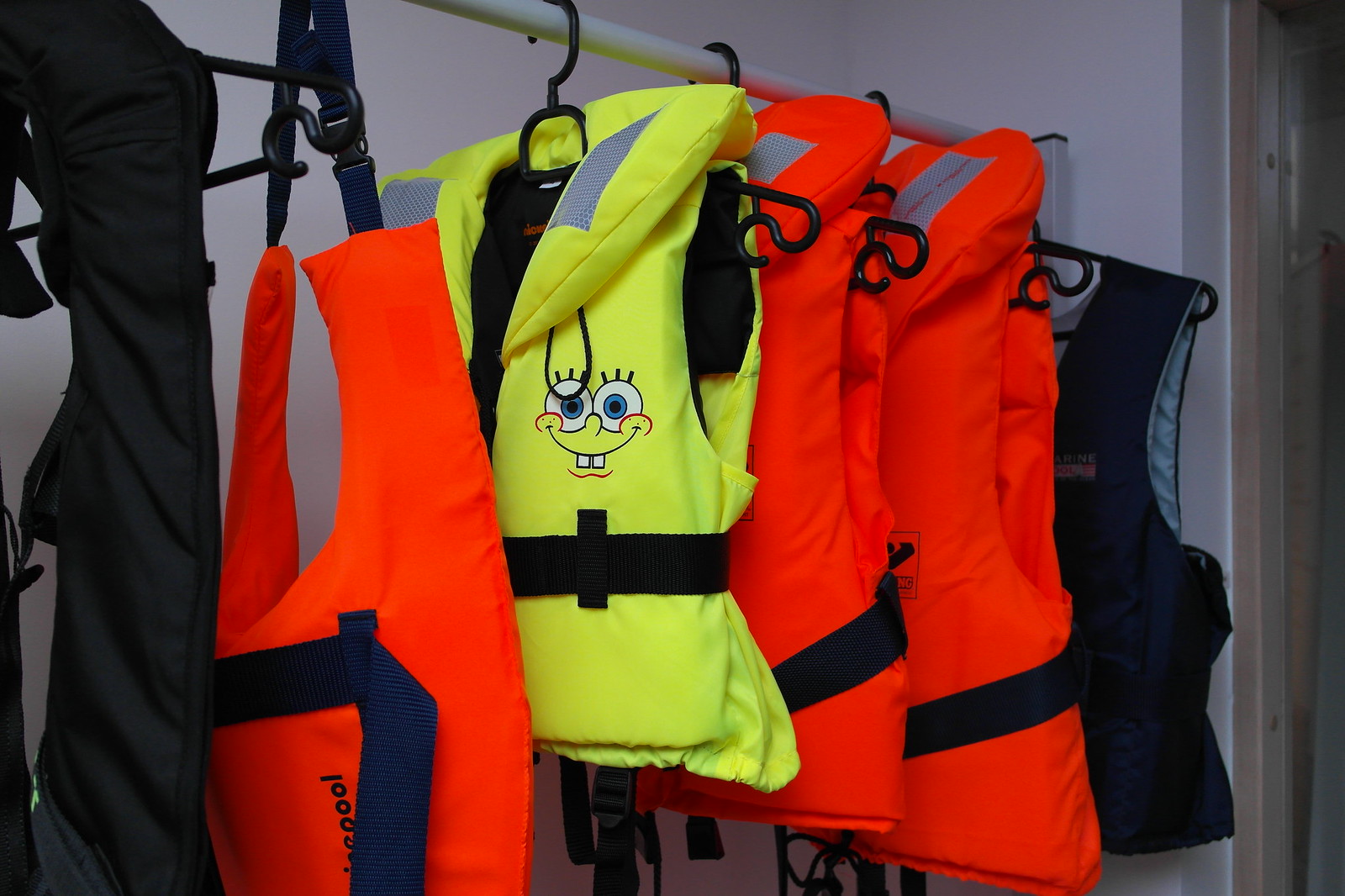The image depicts a group of life jackets hanging on a metallic post, likely on a boat. Among them are three bright orange life jackets with partially obscured text due to the straps. There is also a distinctive yellow life jacket featuring Spongebob's face, which is notably smaller and likely intended for children. Additionally, there is one black life jacket. All of these are suspended on black hangers. The backdrop includes a doorway with a metallic frame and a pale purple or lavender wall. The post extends horizontally between the visible wall and another out of sight. Other parts of the boat are faintly discernible in the background.